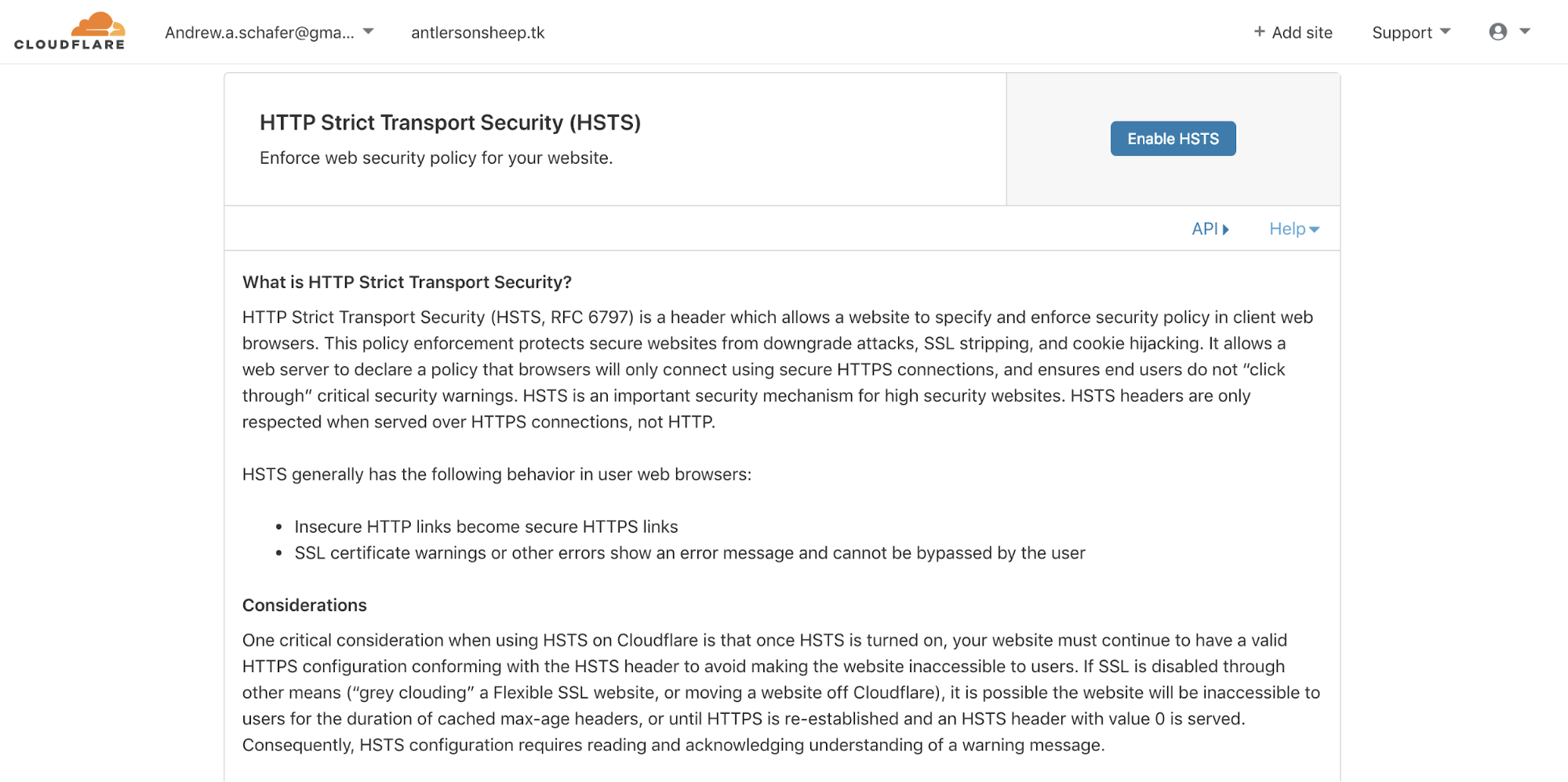The image displays a Cloudflare interface, highlighting various elements related to web security settings. On the left side, there is a partially obscured email address "andrew.a.shaffer at Gmail" shown as "gma.dot....". To the right of the email, there's a "plus" icon possibly associated with site support. The profile section features a blank profile icon.

Prominently displayed is the section related to HTTP Strict Transport Security (HSTS). The heading "Enable HSTS" is presented in a blue rectangle with white text. Below it, the description reads, "Enforce web security policy for your website." Within this description, there is a brief explanation of what HSTS entails: "HTTP Strict Transport Security (HSTS) is defined in RFC 6797 and is a header that allows a website to specify and enforce security policy in client web browsers."

The image overall illustrates the options and settings available in the Cloudflare interface for enhancing web security through HSTS.